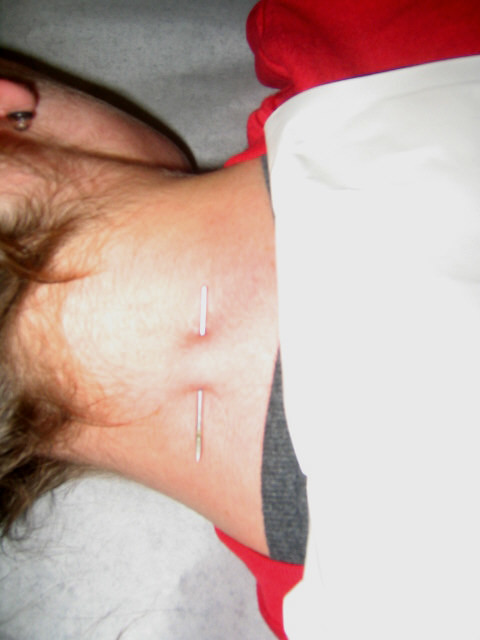The image is a color photograph, slightly rotated, capturing a detailed view of the back of a person's head and neck. The individual, likely male, has short brown hair ending just above the nape. His right earlobe is visible, adorned with a thick plug piercing. He is dressed in a blue jacket with red collar and sleeves, over a partially visible white shirt. The setting gives a clinical feel, with a white sheet suggestive of a doctor's office. Centered in the composition is a disturbing sight: a thick, silver needle, possibly rusted at the tip, which pierces through the pinched skin at the back of his neck in a manner reminiscent of crude acupuncture or a horrific body modification. The immediate area around the needle appears to be non-bleeding, though the implication is it might have bled previously. The focus is sharp, intensely zoomed in on the unsettling needle, accentuating the tension and discomfort of the scene.